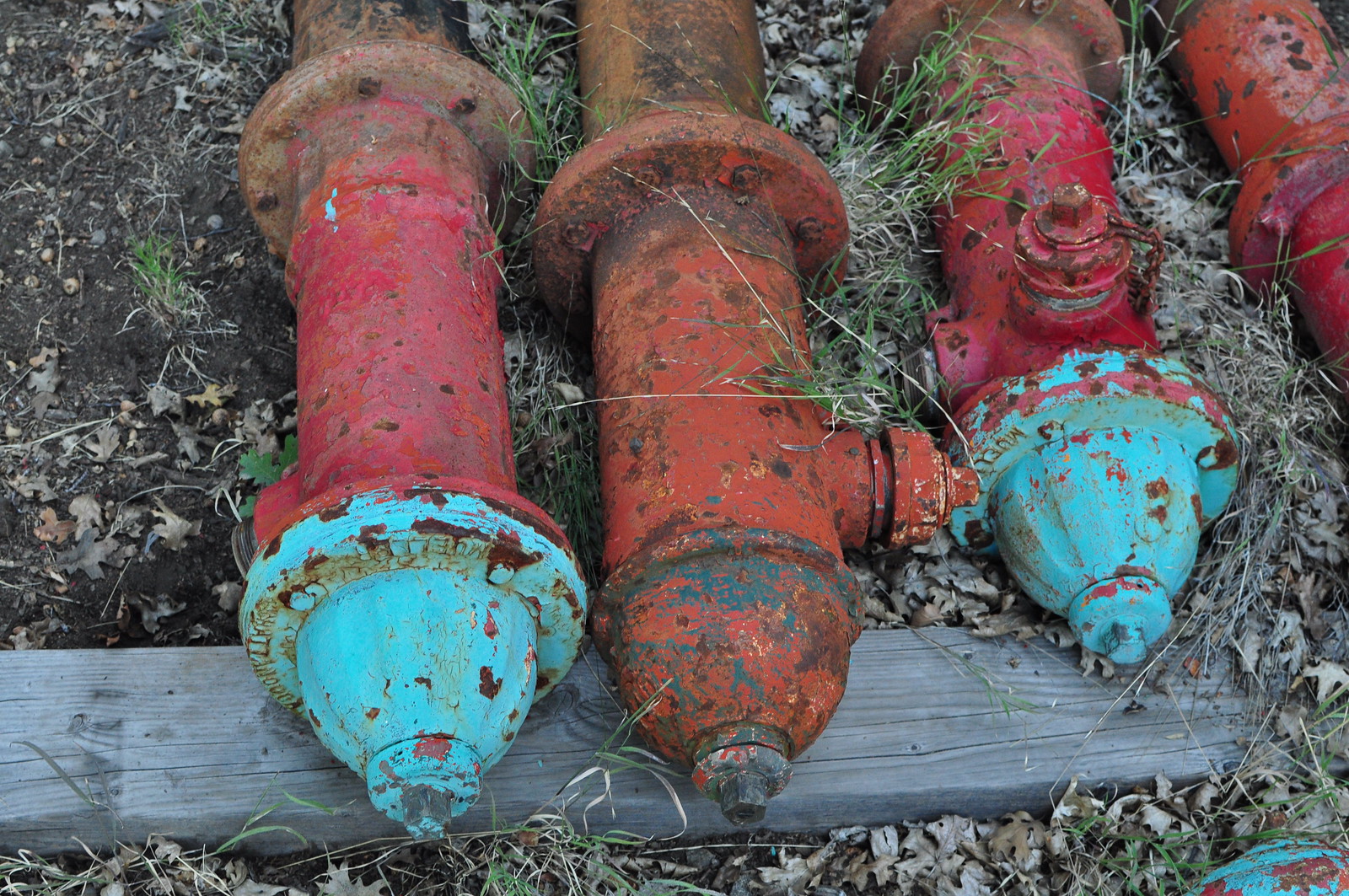This photograph depicts four old, rusted fire hydrants lying horizontally on a patchy dirt surface strewn with dead brown leaves and occasional tufts of grass. Predominantly red, two of the hydrants feature bright blue tops, contrasting with their heavily corroded bodies. These hydrants are laid side by side, with the tops resting against a worn gray 2x4 wooden plank at the bottom of the image. The hydrants' chipped paint and extensive rust damage suggest they are well past their prime and no longer in service. The scene evokes an atmosphere of abandonment, with the hydrants seemingly discarded and surrounded by neglect.